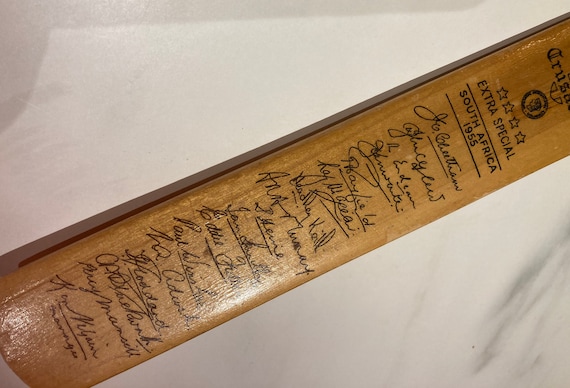This color photograph, captured in landscape orientation, showcases a vintage collector’s edition signed cricket bat. The bat, made of brown wood, stretches diagonally from the top right corner to the bottom left corner, set against a creamy white background. Measuring approximately one foot in length and a couple of inches in depth, the bat features intricate details. At the top, there is a partially visible logo with four stars and the phrase "Extra Special" engraved underneath. Directly below, the text reads "South Africa 1955." The lower portion of the bat is adorned with approximately 15 signatures from notable cricket players of that era, elegantly signed in black ink. The overall photographic style is realistic, emphasizing the bat’s historical and collectible significance.